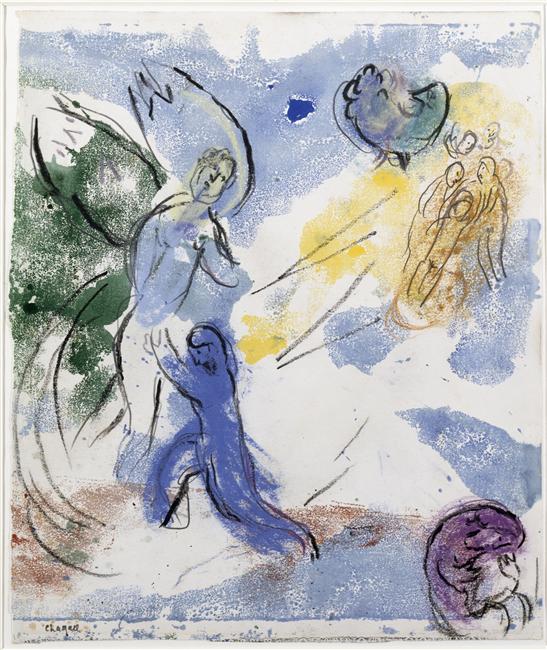The image is an abstract, hand-drawn piece featuring a variety of colors and rapid, erratic strokes. Dominating the center-left, a large humanoid figure, mainly in dark blue, adopts a dynamic pose with one leg stretched out behind and the other to the side, facing left. This figure's left hand pushes against a lighter blue, seemingly ethereal female character above, featuring long, flame-shaped hair and a concerned expression. This woman appears to be drifting or floating to the right, with traces of the wind replacing her leg.

Behind these central characters are splotches of green, likely suggesting trees, while black motion lines give the piece a sense of frenetic energy. To the right, a cluster of brown-colored figures engage in what could be interpreted as pushing or embracing each other. Above them, a large, puffy cloud transitions from bluish on its left half to more green-blue on its right. The bottom right corner features a bird or chicken-like figure, with purplish hair covering its head and simplistic round hands without fingers. This intriguing and multi-faceted artwork uses a predominantly white background, interspersed with smudges of colors like blue, yellow, green, and red, creating an overall impressionistic and vibrant scene.